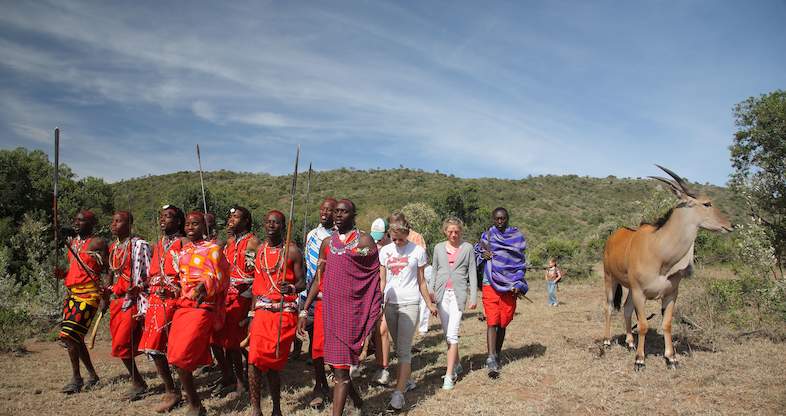The photograph, rectangular in shape, captures an outdoor scene under the bright midday sun in a hot, semi-arid environment. The ground and grass appear yellow and dried out, suggestive of a prolonged dry spell. The backdrop reveals rolling hills adorned with sparse vegetation and a striking blue sky punctuated by fluffy white clouds.

Dominating the center of the image is a vibrant scene featuring a group of African tribespeople. These individuals, dark-skinned and muscular, are adorned in bright red traditional clothing, with one person draped in a blue blanket. Most hold tall, metal spears. Interspersed among them are two Caucasian females dressed in modern Western attire, specifically white t-shirts and capri pants, emblematic of tourists or visitors. In the mix is a large animal resembling an ibex or possibly an antlered cow, characterized by its brownish back and white front, suggesting a creature that could be ridden.

The scene conveys a sense of cultural juxtaposition, with the traditional attire and spears of the African tribespeople standing in stark contrast to the casual, everyday clothing of their Western companions. Adding to the complexity are hints of a smaller child walking amidst the group, contributing to the dynamic and communal atmosphere of the scene. The overall effect is one of beauty and intriguing cross-cultural interaction, set against a picturesque landscape that evokes both the harshness and splendor of the arid terrain.